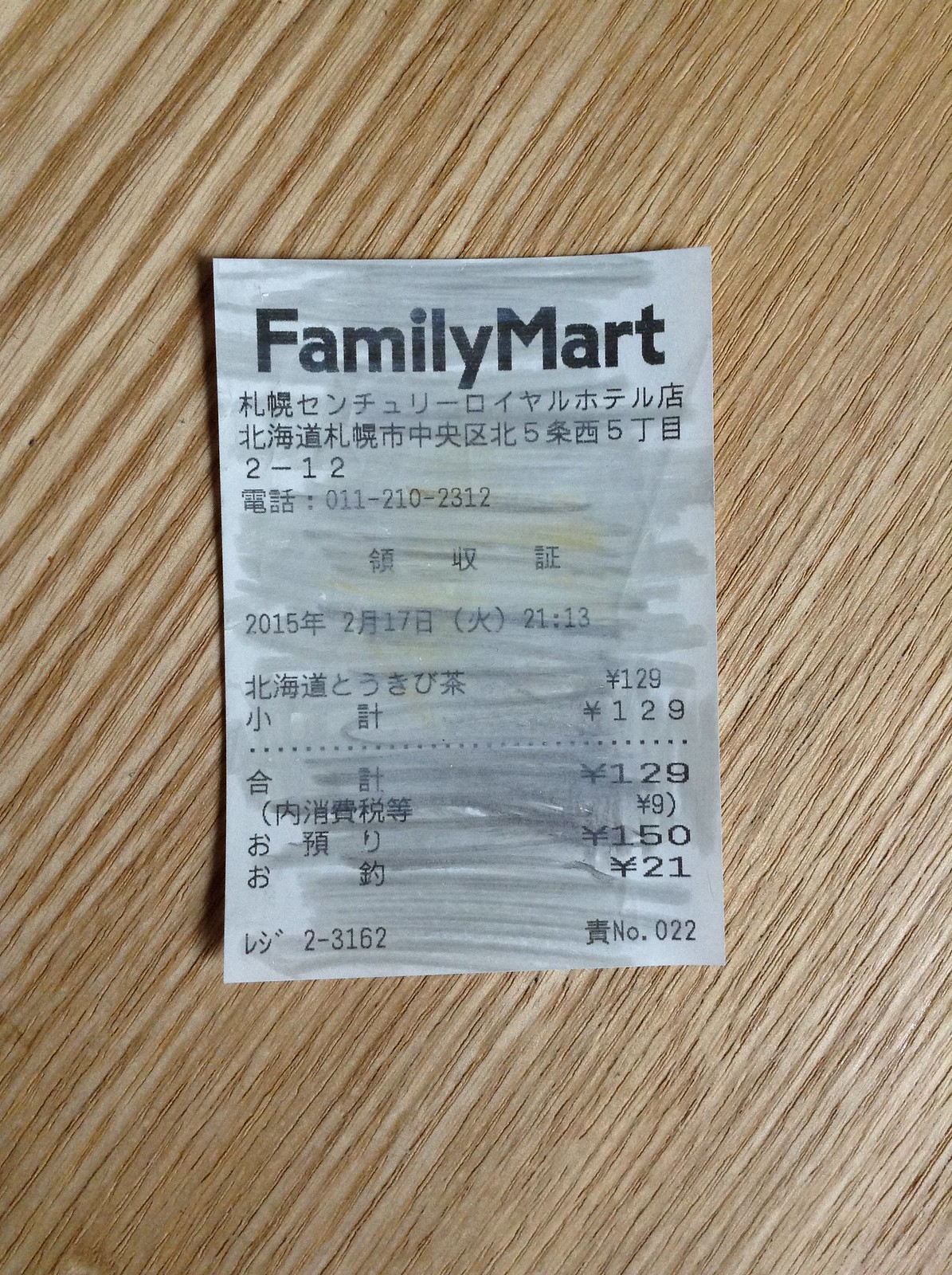The photograph captures a detailed image of a white receipt with black font from "Family Mart." The top of the receipt prominently displays "Family Mart" in English, followed by several lines of text in Japanese. Near the top, there is a sequence "2-12," trailed by a Japanese character and a string of numbers. Below this, more Japanese characters are interspersed with the number "2015," leading to another string of characters, and then "2113." On one side of the receipt, there is an alignment of numbers: "129, 129, 150, and 21." At the bottom, the receipt shows "2-3162" on one side and "022" on the opposite. The receipt is placed on a light wood-grain table with a blond hue, adding a warm, contrasting backdrop to the monochrome receipt.